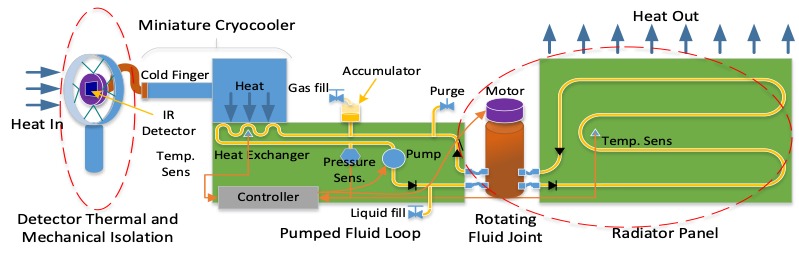The image depicts a detailed scientific diagram of a temperature control system, specifically a miniature cryocooler. On the left side, arrows labeled "heat in" indicate the introduction of heat into the system. The initial section features a "detector thermal and mechanical isolation" and an "IR detector" situated near a "cold finger," which is responsible for channeling heat to a "heat exchanger." The heat exchanger is connected to various components including a "temp sensor," "pressure sensor," "controller," and "pumps." These pumps circulate the heat exchange fluid throughout a fluid loop system. Integral to this system is a "motor" with a "rotating fluid joint," which facilitates fluid movement to a "radiator panel." The radiator panel features multiple temperature sensors and dissipates heat out of the system, indicated by arrows labeled "heat out" at the top right. Additional elements include an "accumulator," a "purge valve," and a "liquid fill pump," ensuring fluid regulation within the loop.